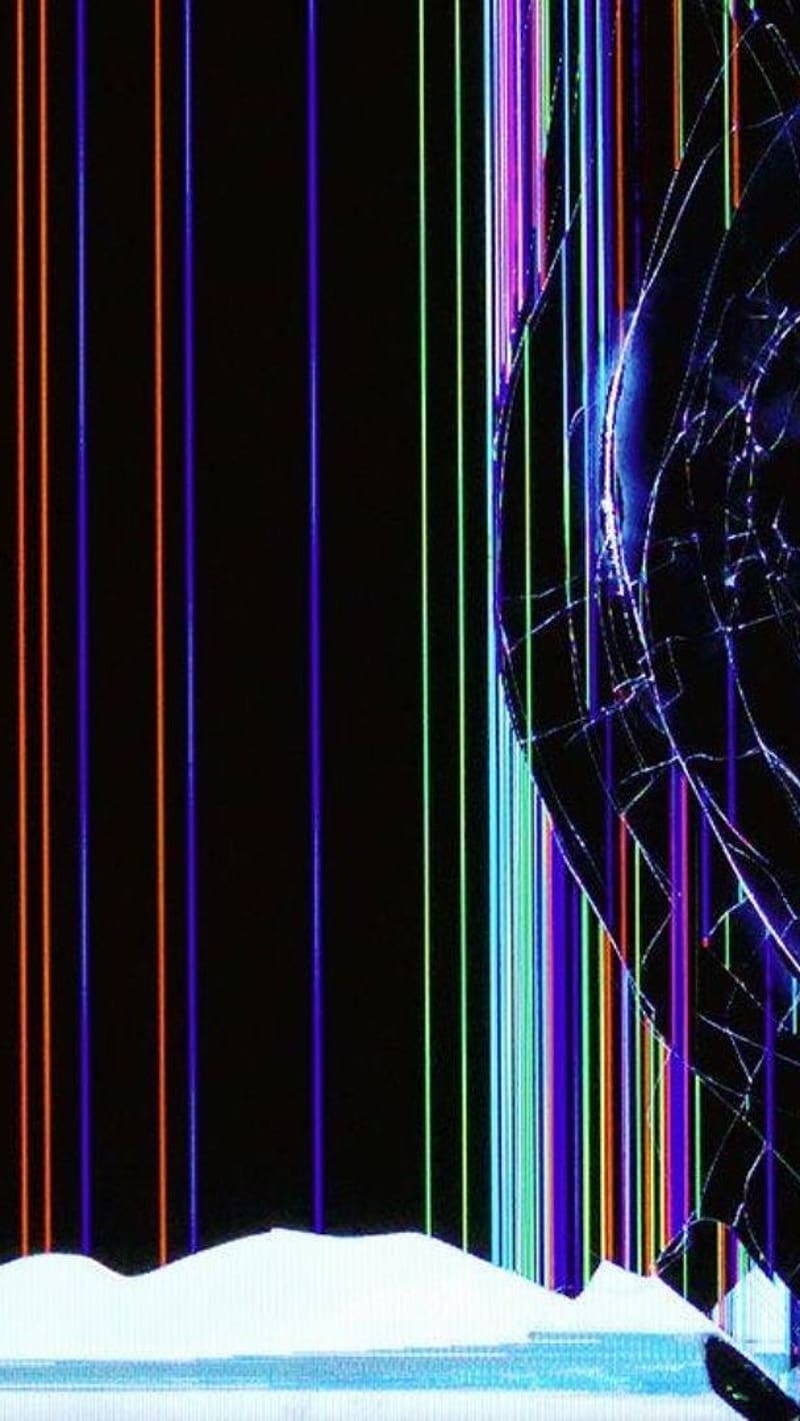The image presents a striking piece of abstract art set against a black background, dominated by numerous vertical lines in vibrant colors including purple, orange, cyan, green, and shades of red. Toward the right side of the image, there is a notable partial circular object resembling fractured glass, highlighted with purple accents and permeated by the vertical lines, which then abruptly stop. This fractured circular element appears illuminated with bright purple and white lights, creating a sense of brokenness or crackling energy. 

At the bottom of the image, a lighter colored section takes up roughly one-fifth of the frame, blending off-white hues with light blue streaks in a jagged pattern that resembles a mountain range or potentially snowy hills. These lower light blue and white areas add a serene contrast to the vivid vertical lines, which are more concentrated and closely spaced on the right side, creating a denser and more dynamic visual effect. The piece as a whole evokes a scientific or spectral feel, leaning heavily on the interplay of shapes and colors rather than depicting a literal scene.